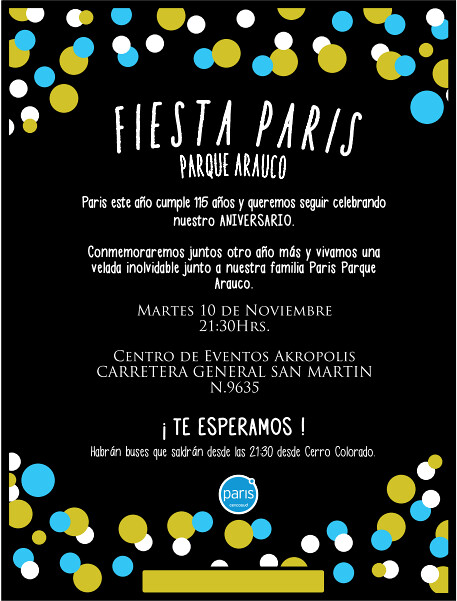This is a computer-generated color poster designed for an upcoming event, featuring a stark pure black background. The entire poster is decorated at the top and bottom with numerous dots of varying sizes and colors, including small white dots, medium blue dots, and larger brown dots, along with some gold elements.

The title "Fiesta Paris" is prominently displayed in bold white letters across the top. Below this, additional text in Spanish reads "París Este Año Cumple 115 Años y queremos celebrando nuestro aniversario." The event is scheduled for "Martes, 10 de Noviembre" at "21.30 hours." 

At the very bottom, a gold bar stretches across the center, approximately 20% width in each direction, providing a subtle accent. Alongside more Spanish text, it mentions the location as "Parque Arauco" and possibly detailed further with "Centro de Eventos Acapulcos, Carrieta General Sin Morten, 9635." The poster concludes with "Te Esperamos" as an inviting final line.